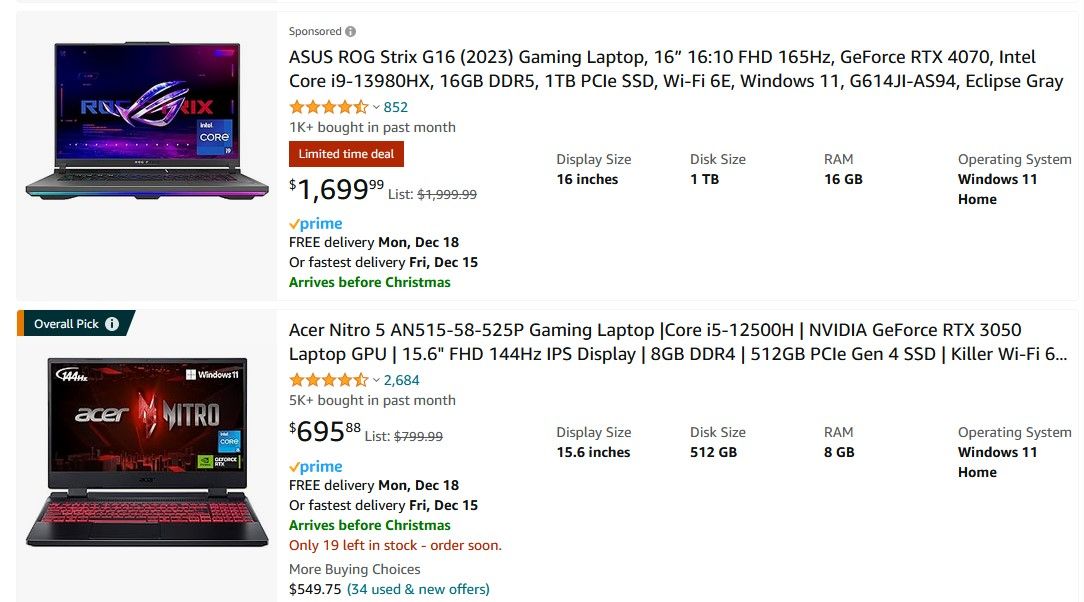The image in the top left corner features a vibrant display of a laptop screen with text in various colors: black, blue, and red, and a purple area in the center. To the right of the screen, the laptop is described as the "ASUS ROG Strix G16 Gaming Laptop" highlighted within a red square that denotes a "Limited Time Deal." The price listed below is $1,699.99. An orange checkmark and blue "Prime" logo indicate its eligibility for Prime services, with green text below stating "Arrives before Christmas."

Beneath this description, there is another section for the "Overall Pick," showcasing the "Acer Nitro Gaming Laptop" priced at $695. This laptop is also Prime eligible, accompanied by the same orange checkmark and blue Prime logo, and the promise of arrival before Christmas in green text. Bold red text alerts potential buyers that there are "Only 19 left in stock, order soon." Further, "More Buying Choices" are listed at $549.75, with blue parentheses mentioning "34 used and new offers."

To the right, additional specifications for the Acer Nitro Gaming Laptop are provided: a display size of 15.6 inches, a disk size of 512 gigabytes, and 8 gigabytes of RAM.